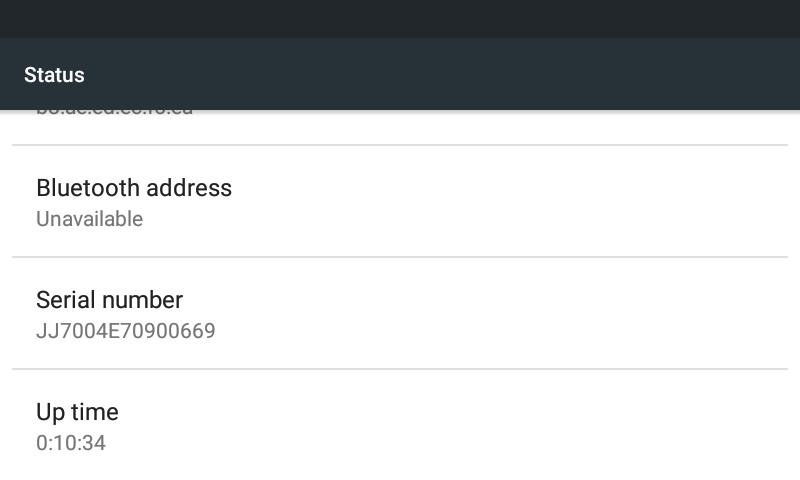This image is a screenshot from a website displaying various device details in a structured format. At the very top, there is a horizontal black status bar labeled "Status." Directly beneath the status bar, there is a category labeled "Bluetooth Address," which displays the value "Unavailable," suggesting that the device's Bluetooth is either disabled or not present. The next category, titled "Serial Number," contains a specific serial number: "JJ7004E70900669." Following this, there is a category labeled "Uptime," which shows the device has been active for "0 hours, 10 minutes, and 34 seconds." The image likely depicts an attempt to set up or check details of a device, possibly during the initial stages of connecting to a Bluetooth network.